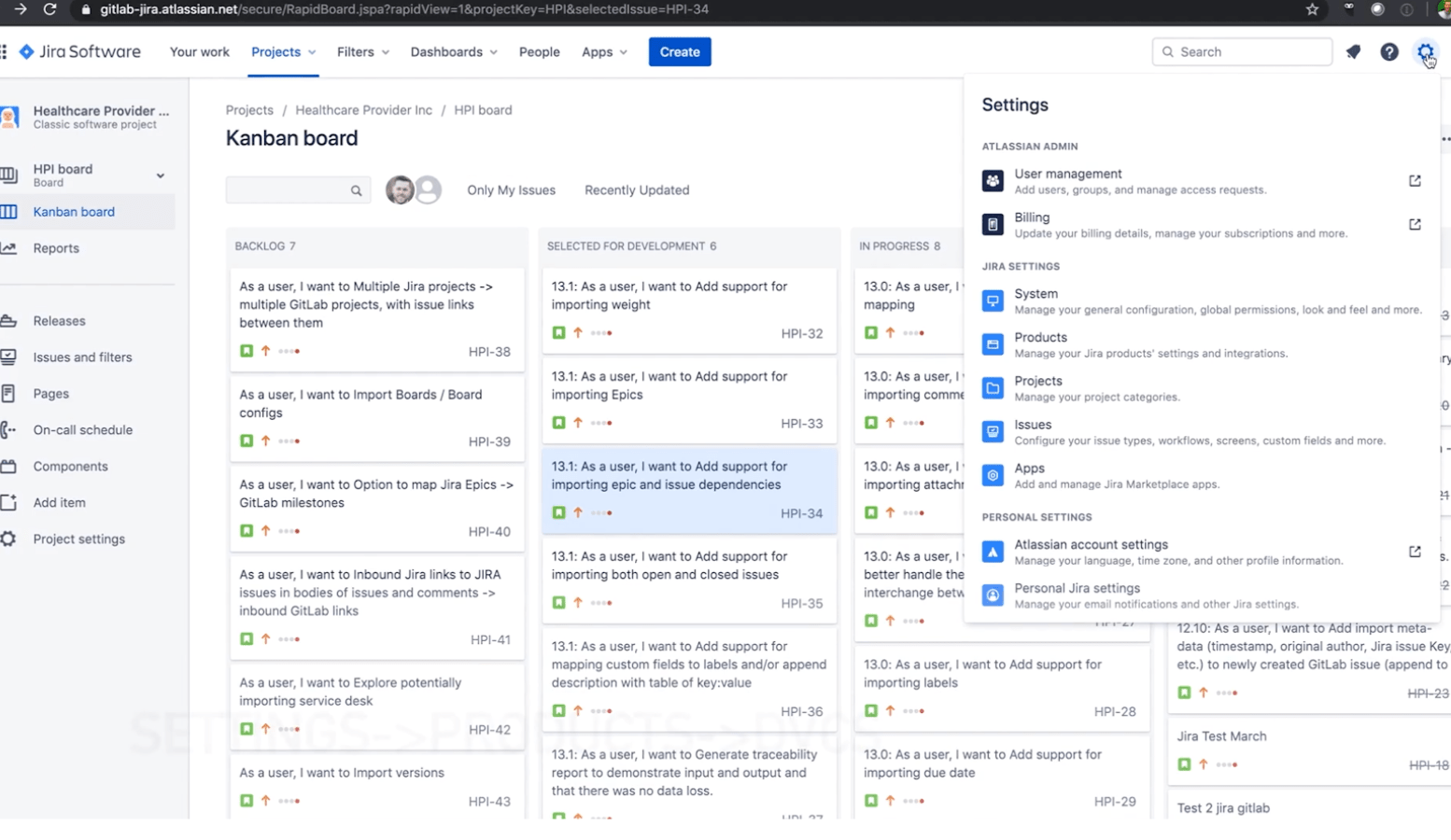This is a screenshot of a Jira Software webpage, specifically tailored for a healthcare provider's project management. The header includes several tabs: "Your Work," "Projects" (currently open and featuring a drop-down menu), "Filters" (with a drop-down menu), "Dashboards" (with a drop-down menu), "People," "Apps" (with a drop-down menu), and a "Create" button. 

On the left sidebar, there are various navigation options listed: "HPI Board," highlighted in blue as the current selection, followed by "Reports," "Releases," "Issues and Filters," "Pages," "On-call Schedule," "Components," "Add Item," and "Project Settings."

The main content area displays the projects for "Healthcare Provider Inc.," with a focus on the "HPI Board" tab. This section features a Kanban board interface with several task cards, though the text on these cards is too small to read clearly. There is also a search box, a user photograph, and a user icon, with filters for "Only My Issues" or "Recently Updated."

An overlay pop-up settings box appears over the task cards on the right side, displaying options such as "Admin," "User Management," "Billing," "Jira Settings," "System," "Products," "Projects," "Issues," "Apps," "Account Settings," and "Personal Jira Settings."